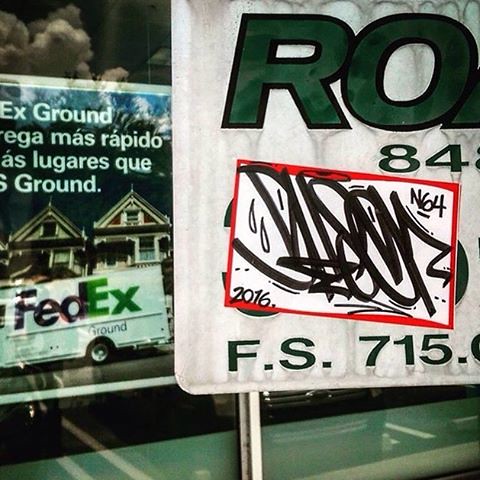The digital photograph, taken outside at night, depicts two advertisement signs on a window. The top portion of the image includes a reflection of a very white, fluffy cloud. 

In the bottom portion of the photo, there's a FedEx sign featuring a white FedEx vehicle with the recognizable logo in blue ("Fed") and orange ("Ex"). Below the logo, small text in blue reads "Ground," and the ad includes Spanish text in white symbols.

Adjacent to the right is a noticeable, large white sign with evident dirt streaks from prolonged outdoor exposure. The sign features green bubble font text saying "RO," followed by "8-4" in black. Additionally, there's a "Hello My Name Is" sticker with a white interior and red border, with "N64" written in black in the upper-right corner. Below, black scribbles and a "2016." text are visible. The main sign also displays "F.S. 715." with part of a number that's not completely readable.

In the reflection, the image captures row houses or townhouses behind the FedEx truck, further enhancing the urban nighttime scene.